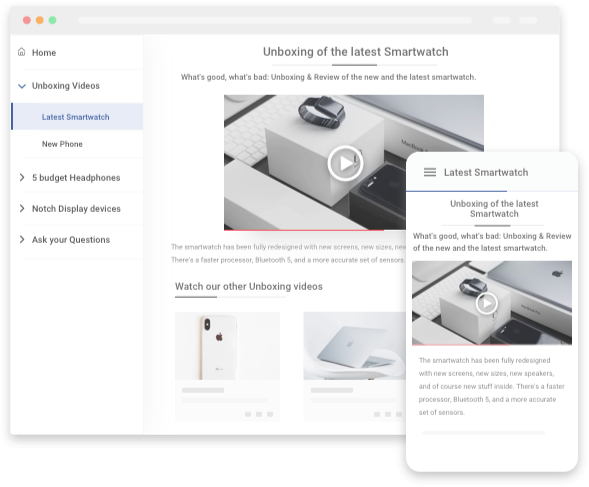Here are two images capturing different devices displaying a webpage and a related screenshot.

1. **Web Browser on Apple MacBook:**
    - The web browser window shows the typical macOS interface with three colored circles (red, orange, and green) on the top left corner indicating window controls.
    - The webpage title bar features a "Home" tab on the left.
    - Below the "Home" tab is a collapsible section labeled "Unboxing Videos" with a downward arrow, indicating it is expanded.
    - Within this section, the current page is "Latest SmartWatch," highlighted in blue, and surrounded by other topics like "New Phone," "Five Budget Headphones," "Notch Display Devices," and "Ask Your Questions."
    - The "Latest SmartWatch" page features the main title "Unboxing of the Latest SmartWatch," followed by a subheading: "What's good, what's bad, unboxing, review, the new, and the latest smartwatch."
    - Centrally displayed is a video clip with a play button, ready to be watched.
    - Below the video, a secondary headline encourages further viewing: "Watch our other unboxing videos," accompanied by thumbnails of different products.

2. **Screenshot from a Cell Phone:**
    - The screenshot displays a similar webpage interface adapted for mobile viewing.
    - At the top is the title "Latest SmartWatch."
    - It carries the main headline "Unboxing of the Latest SmartWatch" followed by a video clip with a play button beneath.

Both images illustrate the same "Latest SmartWatch" unboxing content, with the primary image being a detailed web browser view and the smaller screenshot providing a mobile-friendly version of the same page.